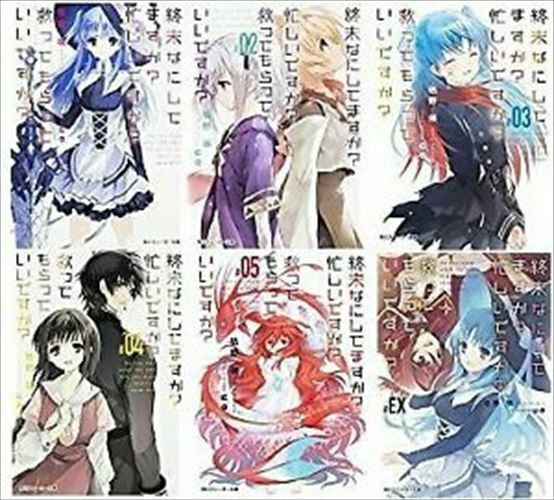The image is divided into six equal sections, arranged in a 3x2 grid. Each section features a distinct anime character or pair of characters, accompanied by Japanese text in the background and labeled with numbers 1 through 6. 

In the top left section, labeled 1, there is a young woman adorned in a hat and pinafore dress, resembling a maid outfit. The top center section, labeled 2, depicts two anime characters standing back-to-back; the character on the left wears a purple dress while the one on the right dons a tan and brown dress. The top right section, labeled 3, showcases a cheerful female character with blue hair, wearing a scarf and black dress, facing forward.

Moving to the bottom row, the bottom left section, labeled 4, presents another pair of back-to-back characters. In the foreground is a girl with large eyes and dark brown hair facing forward, while behind her is a man in a black jacket looking to the right. The bottom center section, labeled 5, features a character with long flowing red hair, whose upper body is partly visible, and a fish image floating above her head. Finally, the bottom right section, labeled 6, portrays a blue-haired female dressed in a blue outfit and white skirt, with a large bow-tied bonnet.

The overall layout and design give the impression of postage stamps, each square matching up precisely in size and style.